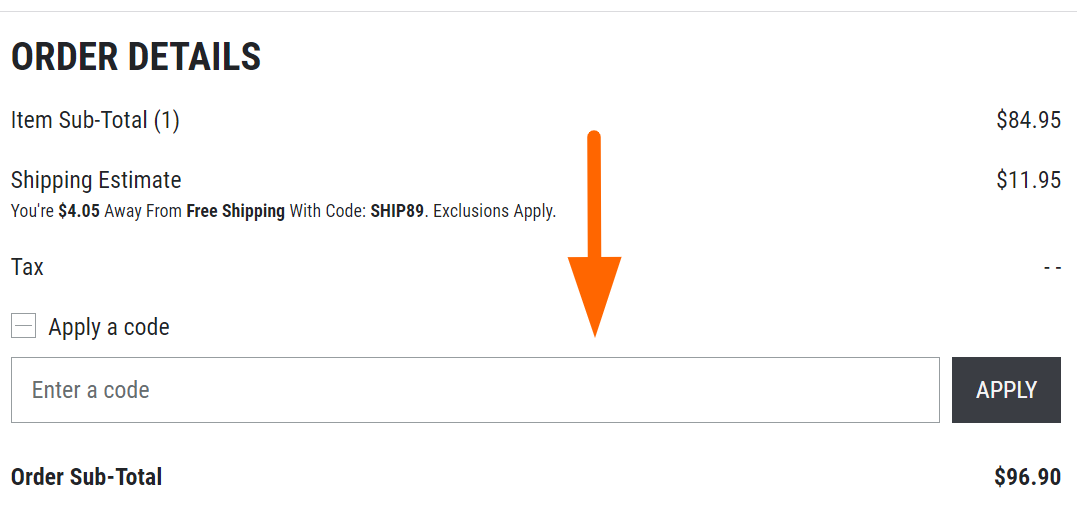This image is a screenshot capturing the details of an online order summary. Set against a clean white background with crisp, black fonts, the layout begins with the heading "Order Details" at the top. Just above this heading, a thin gray line is visible, subtly dividing the header from the content below.

Below "Order Details," the screen lists the breakdown of costs. The item subtotal, noted within parentheses as (1), is priced at $84.95. Following this, there is an important notification about shipping: “You’re $4.05 away from free shipping with code SHIP89, exclusions apply.” The standard shipping fee without the code is $11.95.

Moving down, there is a section for tax, marked by two black dash marks crossing horizontally. Adjacent to this, there is a prompt to apply a code, highlighted by an orange arrow pointing towards a long rectangular input box outlined in black with a subtle minus sign embedded in it.

Next to this input box is a gray box with the word "Apply" printed in white. Both boxes are designed for easy interaction within the order process.

At the bottom of the image, the order subtotal stands at $96.90, providing a clear and concise summary of the total cost. 

The fonts are large and legible, ensuring the text is easy to read. The image quality is impeccable with no signs of pixelation or graininess, making the details crystal clear. There are no additional objects, text, or elements present within this image to distract from the information presented.